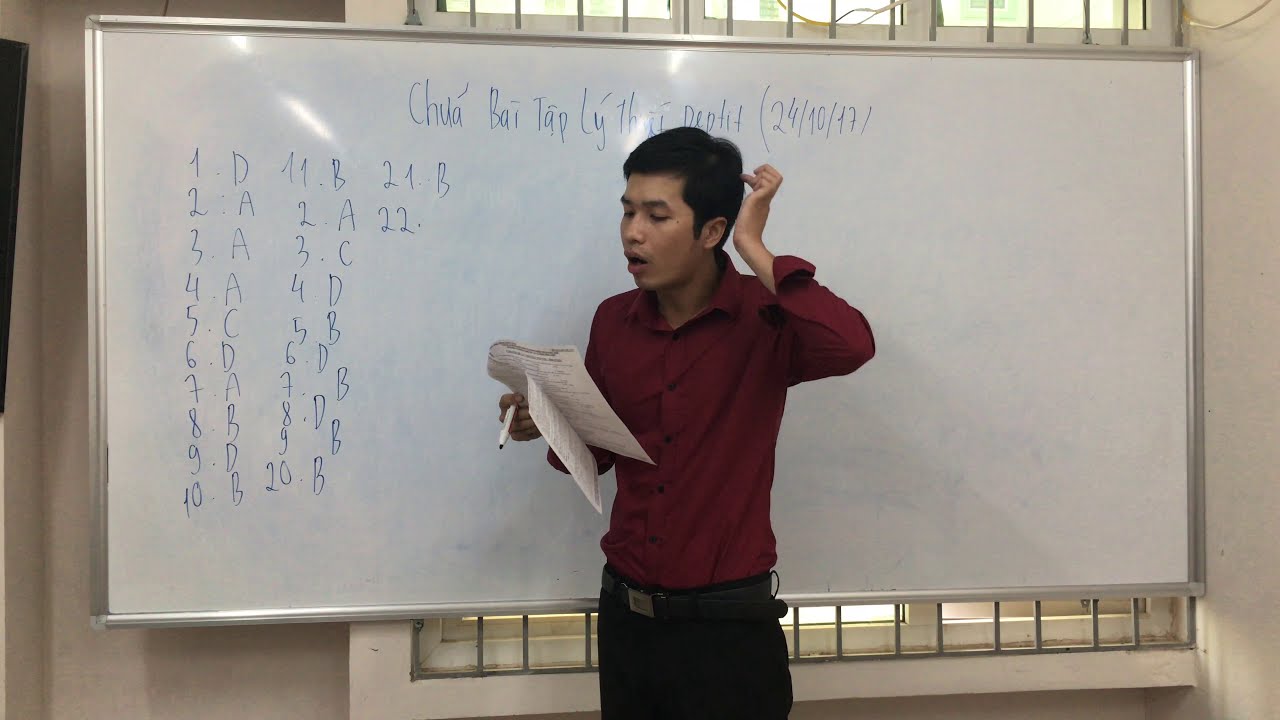In the image, a young Asian man stands in front of a large rectangular whiteboard, appearing to teach a class. He has short dark hair and is dressed in a burgundy button-up shirt paired with black pants and a black belt. Positioned centrally in the frame, he adopts a three-quarter profile stance, facing slightly to the left. In his right hand, he holds a couple of papers and a pen, while his left hand is raised, scratching the back of his head with a finger, giving him a somewhat confused look. His mouth is partially open as he looks down at the papers he is holding. 

The whiteboard behind him contains blue lettering in a foreign language, possibly Japanese or Chinese, along with numbers and letters arranged in vertical columns. The background features a cream-colored wall with windows framed by vertical metal bars, allowing light to filter through. This setting suggests an academic environment, potentially in China or Japan, where the professor seems to be figuring out the next part of his lesson plan.